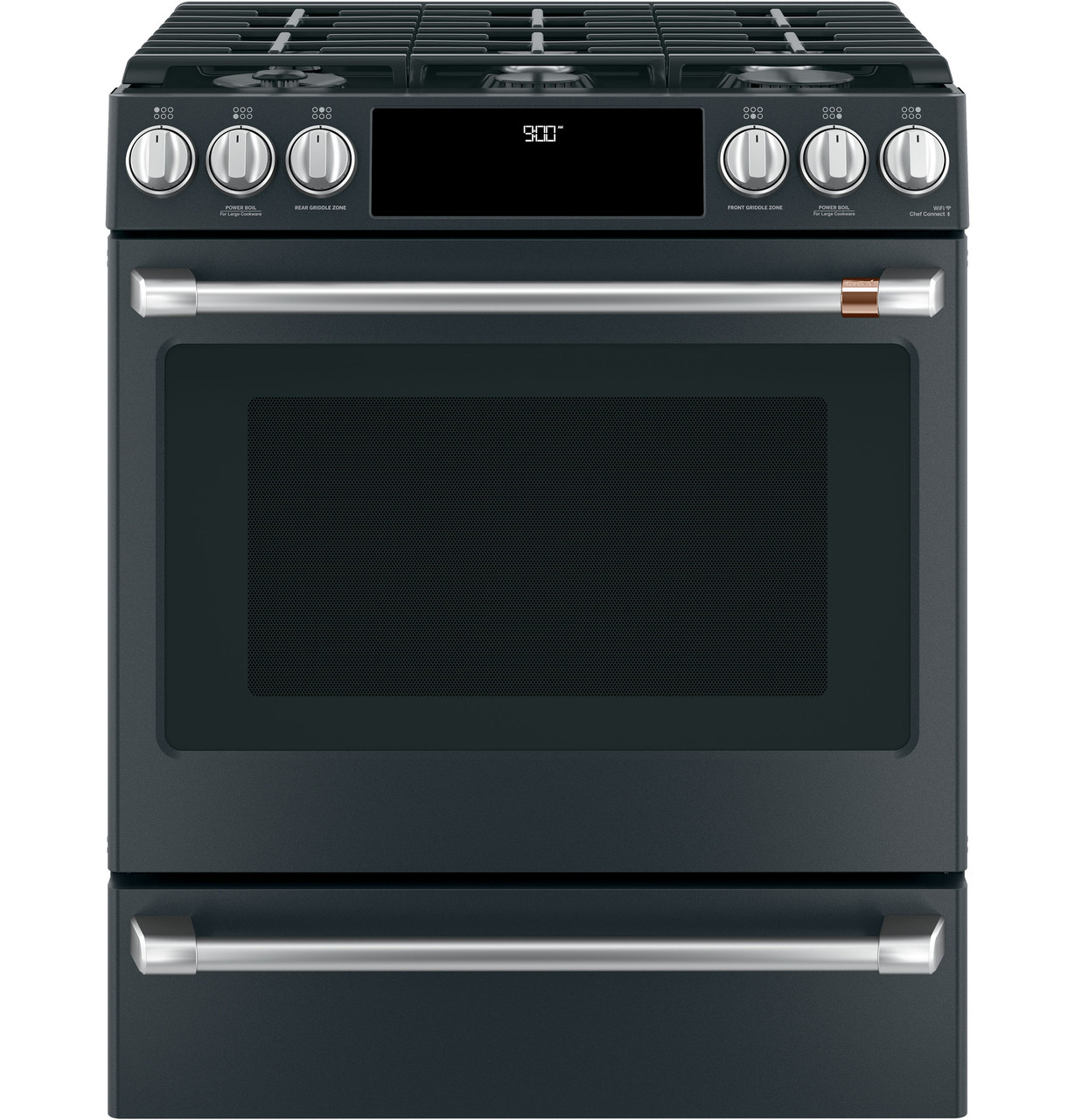The image is a professional product photo featuring a sleek black oven range prominently displayed against a plain white background. The stove has a distinctive layout, including a lower warming drawer and a main oven compartment accessible through a silver handle that has a small gold accent on the end for a touch of elegance. On the top, the range is equipped with six burners, each controlled by a set of silver knobs—three on the left and three on the right side of the front panel, totaling six knobs. The front of the stove displays the time, set at 9 o'clock, in bright digital digits, indicating its digital interface. The stovetop features continuous grates that cover all the burners. The overall design includes a second silver handle, likely for the broiler section, which is also closed. No brand name or advertisement markings are present, making the focus solely on the appliance itself.